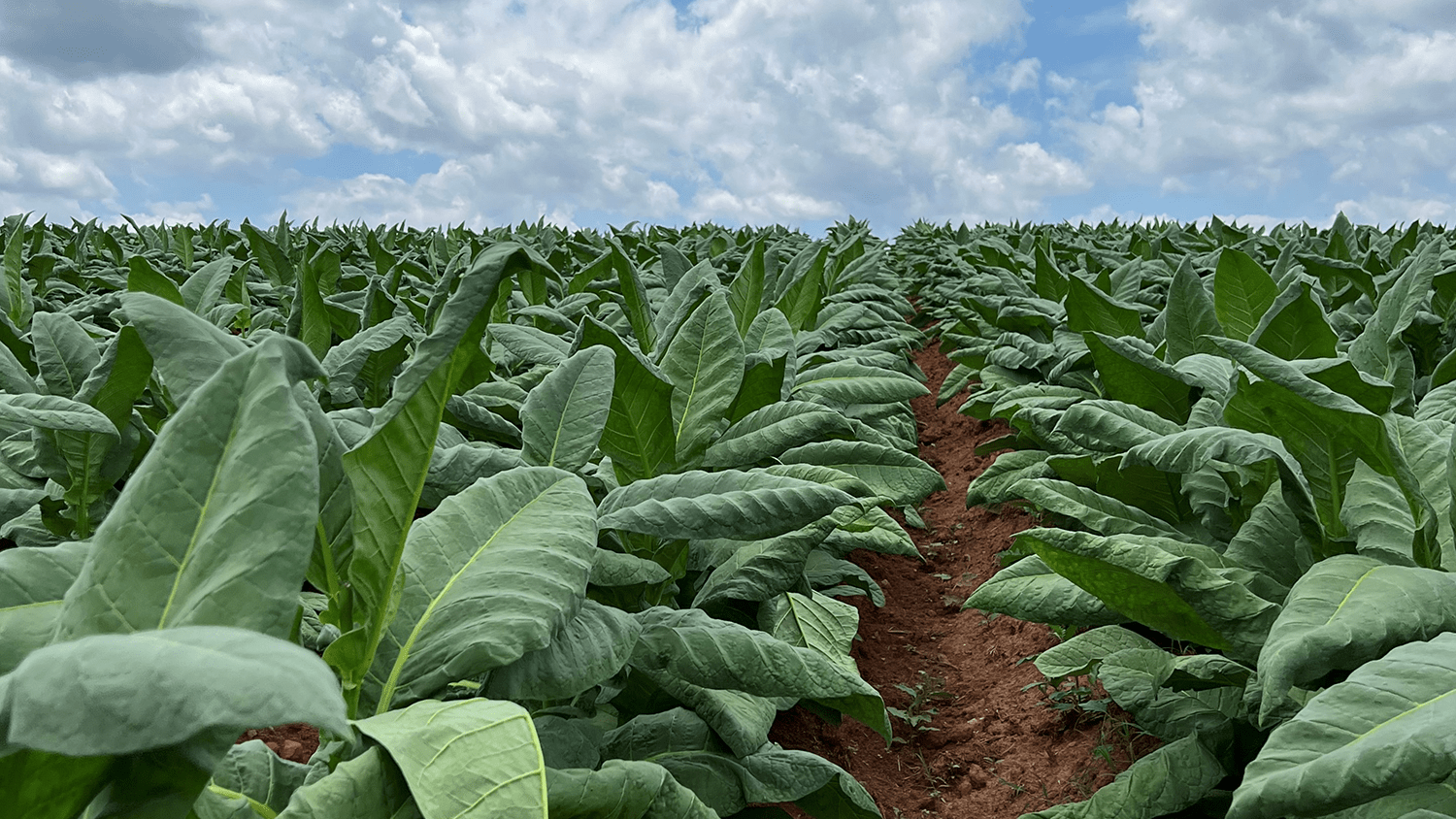This image captures an expansive and lush green field of crops, all uniform in shape and size, filling the majority of the frame with their large, round, and curling leaves. The crops appear healthy and robust, flourishing against a backdrop of deep brown, almost reddish soil. A single dirt row cuts through the field, likely serving as a path for farmers. The scene is bathed in natural daylight, with a wide expanse of blue sky dotted with white clouds stretching across the horizon, occupying about one-fourth of the image. The overall atmosphere suggests a thriving agricultural landscape, teeming with verdant growth under a cloudy, but bright sky.